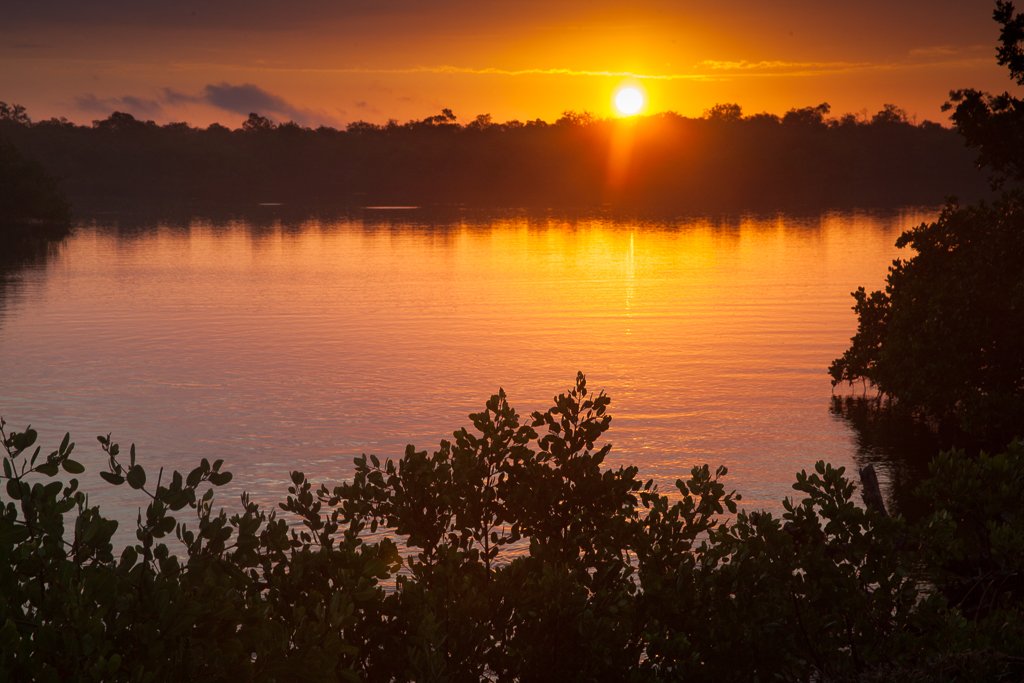The image captures a tranquil sunset over a serene lake. The sky is a stunning gradient, beginning with a bright white sun surrounded by golden yellow hues that fade into orange and then transition into darker shades near the top. Wisps of clouds accentuate the otherwise clear sky. The sun, just about to dip below the horizon, casts a warm glow that creates a beautiful reflection on the calm, glassy surface of the lake, tinting it with shades of orange and purple.

In the background, you see a dense row of trees, their shapes reduced to dark silhouettes against the colorful sky. The horizon is a tapestry of green leaves barely discernible due to the contrast created by the setting sun. The foreground is rich with foliage, depicting a variety of green bushes and shrubs extending across the bottom and up the sides of the image. The greenery in the foreground is dimly lit, their details obscured by the predominant light coming from the sunset.

Overall, the scene exudes a peaceful ambiance, devoid of human presence, focusing solely on the natural beauty and calmness of the landscape. It perfectly encapsulates the serene transition from day to dusk.